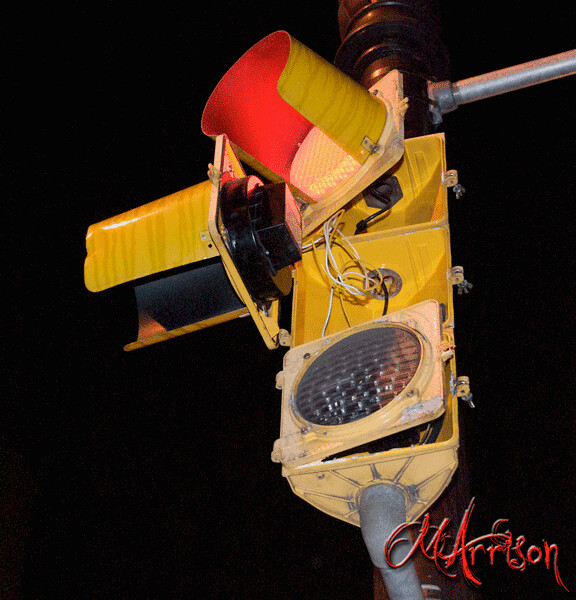The image portrays a deteriorated traffic signal set against a stark black background. The signal's lights are in various states of disrepair, exposing internal mechanisms and wiring. The top light is illuminated in red and its faceplate is ajar at a 40-degree angle. The middle light, also lit but in yellow, dangles open at a 90-degree angle, revealing tangled yellow and white wires as well as a black wire at the top. The bottom light, intended to be green, is unlit and only slightly cracked open at about a 15-20 degree angle. All access doors are hinged on the left. Below the signal, the name "M. Erison" is artistically printed in stylized, swooping red letters with a shadowed black border. The traffic light is affixed to a silver metallic pole and, lower down, a weathered wooden pole, hinting at a possible setting of maintenance or abandonment.